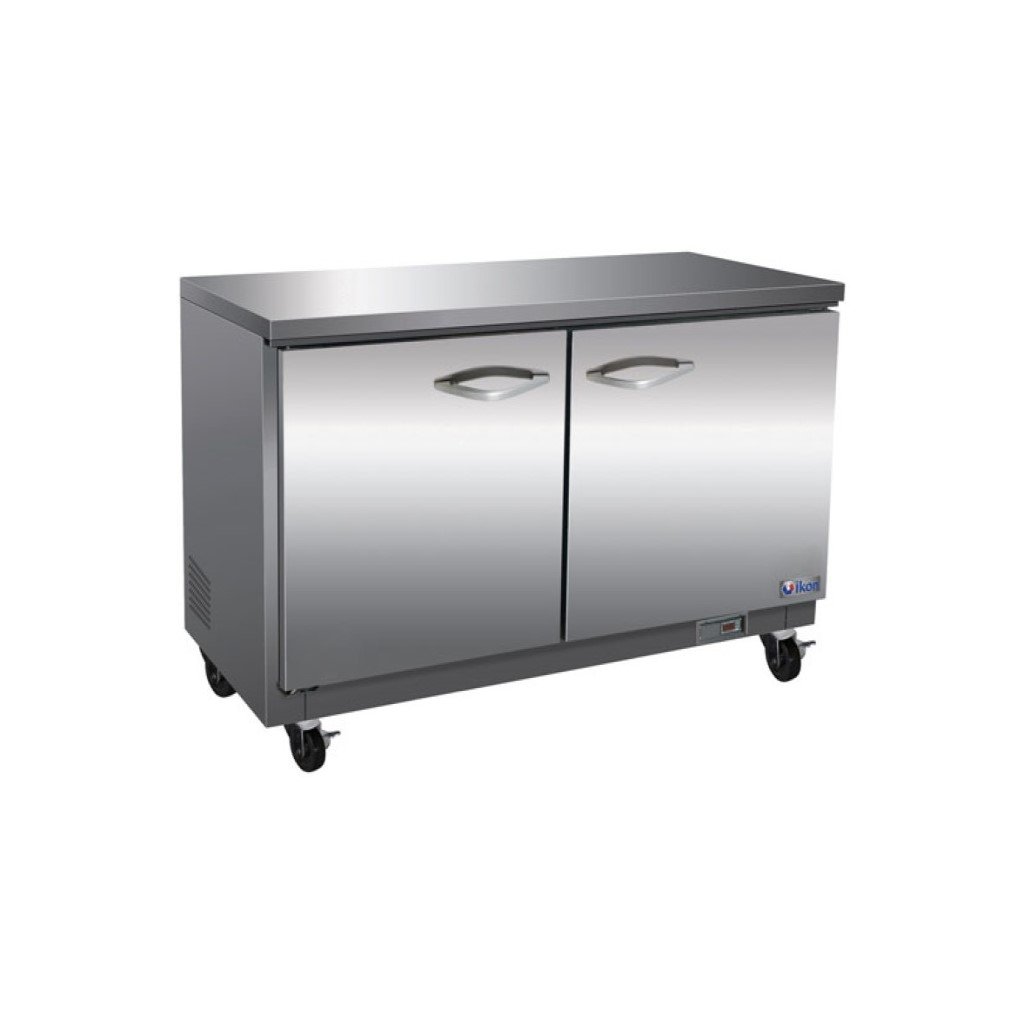The image depicts a commercial stainless steel utility cart with a sleek, shiny silver finish, reminiscent of those used in restaurants. The unit is rectangular and features two front doors with handles in the middle that open outwards, providing access to the stored contents, which could range from food supplies to beverages. The cart is mobile, equipped with four black heavy-duty wheels at the bottom, each featuring brakes to keep the unit stationary when needed. Along the bottom right corner, a small, partially legible brand insignia in red and blue reads "IKON" or "Ikori." On the left-hand side panel, there are vents that suggest it might function as a refrigerated prep table. The top of the cart serves as a durable workspace, potentially lifting up for additional storage access, though this is not entirely clear.